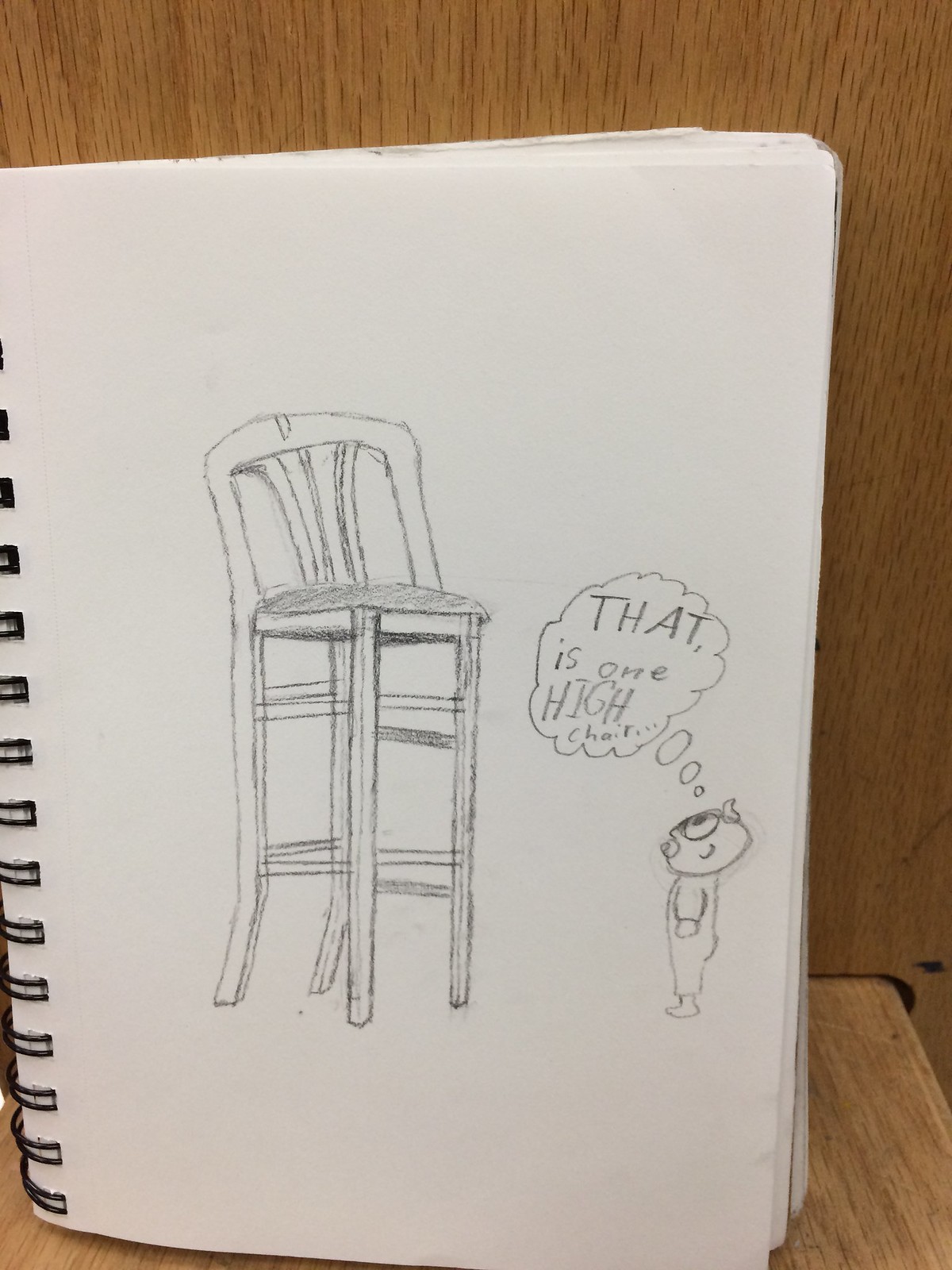This image features an open white-page notebook with a detailed pencil drawing at its center. The drawing, rendered in black pencil, depicts a high chair with long legs and a baby positioned to the right of the chair. Above the baby, there's a speech bubble containing the phrase, "That is one high chair..." The notebook, characterized by its black spirals on the left side, rests on a brown wooden platform. This wooden texture extends to the background wall, providing a cohesive and warm setting for the scene. The drawing is centrally positioned, capturing the viewer's attention amidst the rustic backdrop.